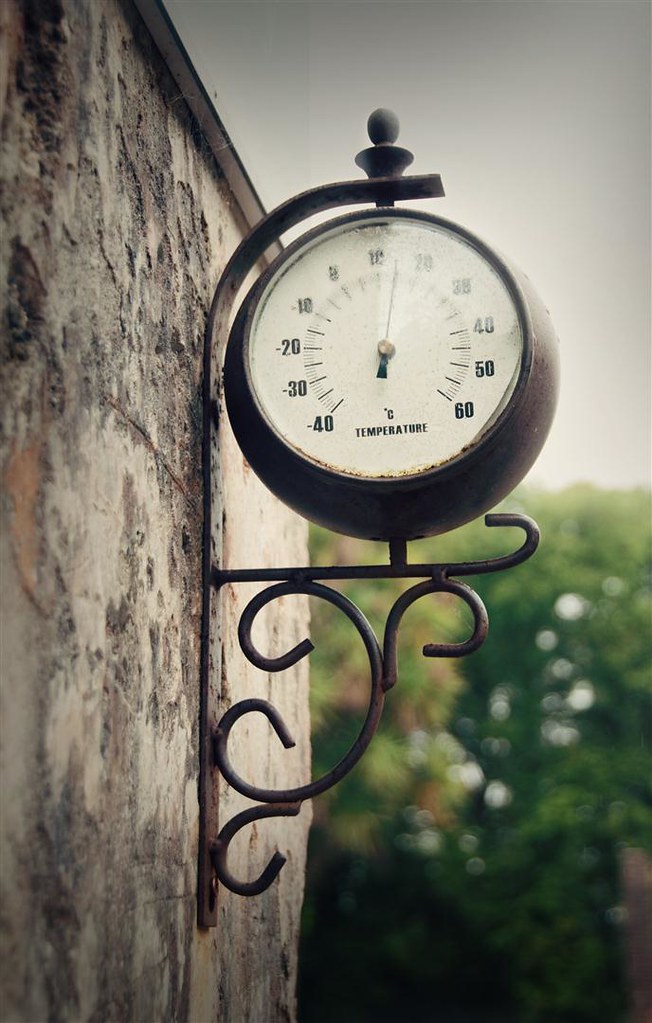A detailed photographic image captures an aging brick building adorned with a decorative iron temperature gauge. The sky is overcast with white and cloudy conditions, yet it remains bright, casting an even light over the scene. In the background, tall, thick trees with vibrant green, yellow, and orange foliage create a blurred backdrop, enhancing the depth of the image. To the right, an out-of-focus brown building can be faintly seen in the distance.

The primary building, close-up and centered in the photograph, is built of gray bricks interspersed with brown rust spots, indicative of its age and weathering. Mounted on its facade is an iron temperature gauge, designed like a clock, with an ornate decorative top and a knob. The gauge projects outward, ensuring it faces directly toward the viewer. The face of the gauge is white, shielded by a glass covering, and it prominently displays the temperature at 15 degrees Celsius.